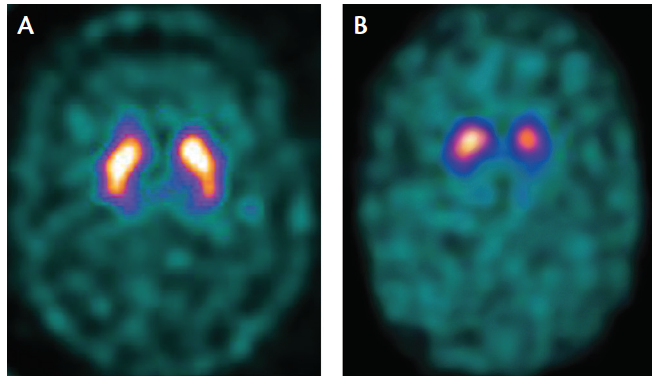The image in question appears to depict two medical imaging scans labeled A on the left and B on the right, both resembling the shape of a human brain. Each image features a prominent mass that primarily glows green, displayed against a black background. Distinct within the mass, there are smaller regions of varying colors—yellow, orange, purple, and blue—highlighting particular details. In image A, these multicolored regions are more pronounced and vibrant, especially in the center, with two bright yellow spots fading to orange, purple, and then blue towards the edges. In contrast, image B exhibits these colored regions in a smaller, less radiant form, suggesting a decrease in intensity or activity. Despite the lack of labels or textual descriptions identifying the specific nature of the scans, the oval, brain-like structures, and the distinctly colored lobes imply some form of brain imaging—possibly illustrating different states or conditions of cerebral activity.